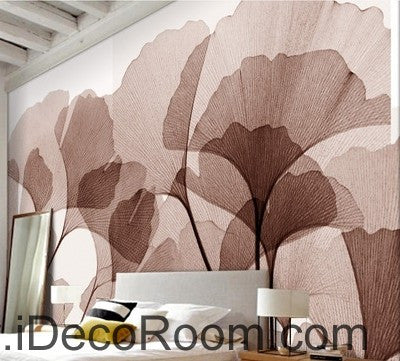This small square image depicts a stylish bedroom setting viewed diagonally. The primary focus is on a feature accent wall adorned with large, overlapping Japanese-style fan flowers in shades of brown and beige, creating a translucent effect that darkens where the shapes overlap. The background of the wall is predominantly a pinkish-brown hue progressing to lighter shades towards the top. Above the featured wall, the ceiling with wooden beams is visible. The image shows the bottom portion of a bed with a white headboard and white linens. To the right, there's a wooden bedside table with a lamp featuring a white drum shade. On the left side, the rest of the wall extends down to the floor. Printed along the bottom of the wall in black lettering is a website address: ".idecorum.com".